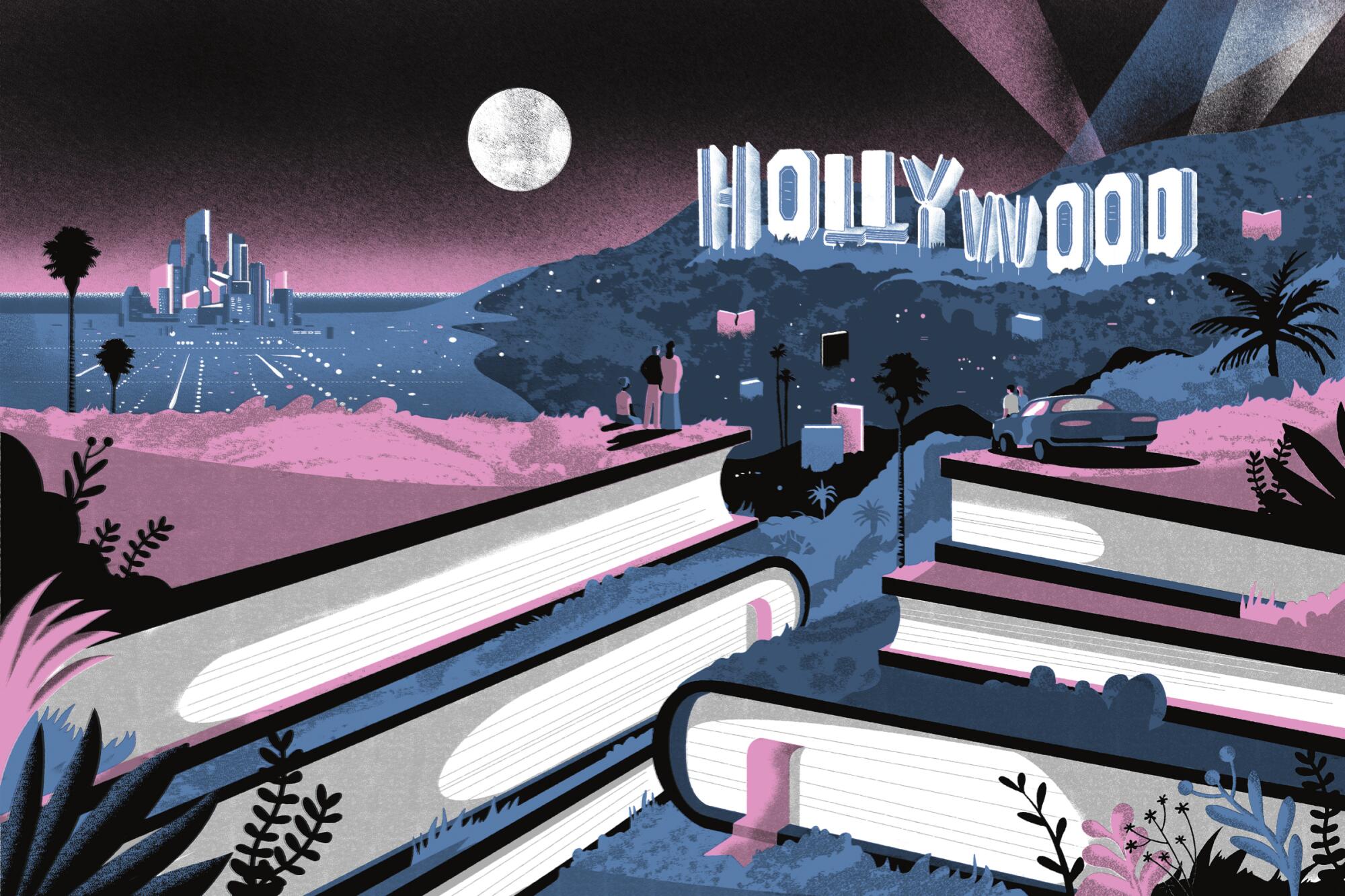This Art Deco-style painting captures a fantastical depiction of the Hollywood Hills and downtown Los Angeles. In the top left corner, the city's imposing buildings rise in the distance, flanked by two palm trees. To the right, the iconic Hollywood sign sprawls across the hills, its letters intriguingly formed from stacked books. Above this, beams of purple, blue, and gray from spotlights pierce the dark purple sky. The scene is dominated by a large, luminous white moon centrally positioned in the sky.

In the foreground, six enormous books of pink and blue hues form a surreal landscape. Three diminutive figures stand atop these books: one person in a pink shirt and blue pants, another in a black shirt and pink pants, and a third individual sitting in a pink shirt. On the right side, a vintage 1950s blue sports car is parked at the edge of the books, aiming toward the Hollywood Hills. Two people sit on the car's hood, gazing out at the view, while a man in a white shirt and blue pants stands nearby. The painting's palette of pinks and blues, coupled with its imaginative elements, imparts a whimsical, old-fashioned flair to this depiction of Los Angeles.